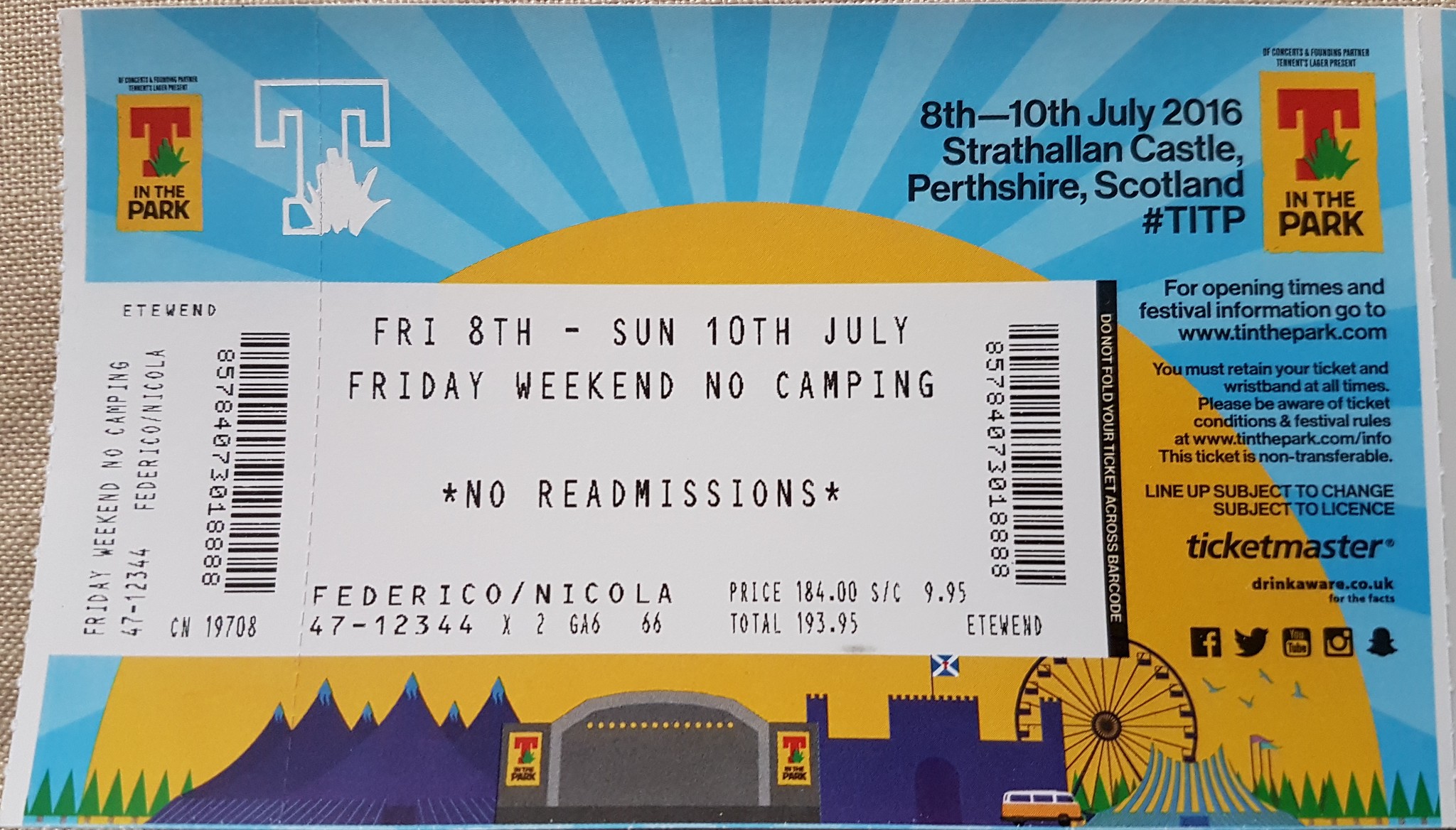The image depicts an event ticket for "T in the Park," held from July 8th to 10th, 2016 at Strathallen Castle in Perthshire, Scotland. The ticket, positioned centrally on a tan fabric background, is overlaid with a picturesque scene featuring a large orange sun with radiating rays, a grand castle, a Ferris wheel, purple tents, and a circus tent. Prominent on the ticket is the event information in black font, detailing "Friday 8th to Sunday 10th July, Friday weekend, no camping, no readmissions." The left-hand side shows the "T in the Park" logo, featuring a red 'T' in a yellow box. Additional text includes festival details, such as "For opening times and festival information, go to www.tinthepark.com," and a reminder to retain the ticket at all times. It also notes that the ticket was purchased for Nicola Federico for $193.95 (inclusive of tax). The vibrant colors in the image include tan, gray, blue, red, yellow, green, black, white, and purple.